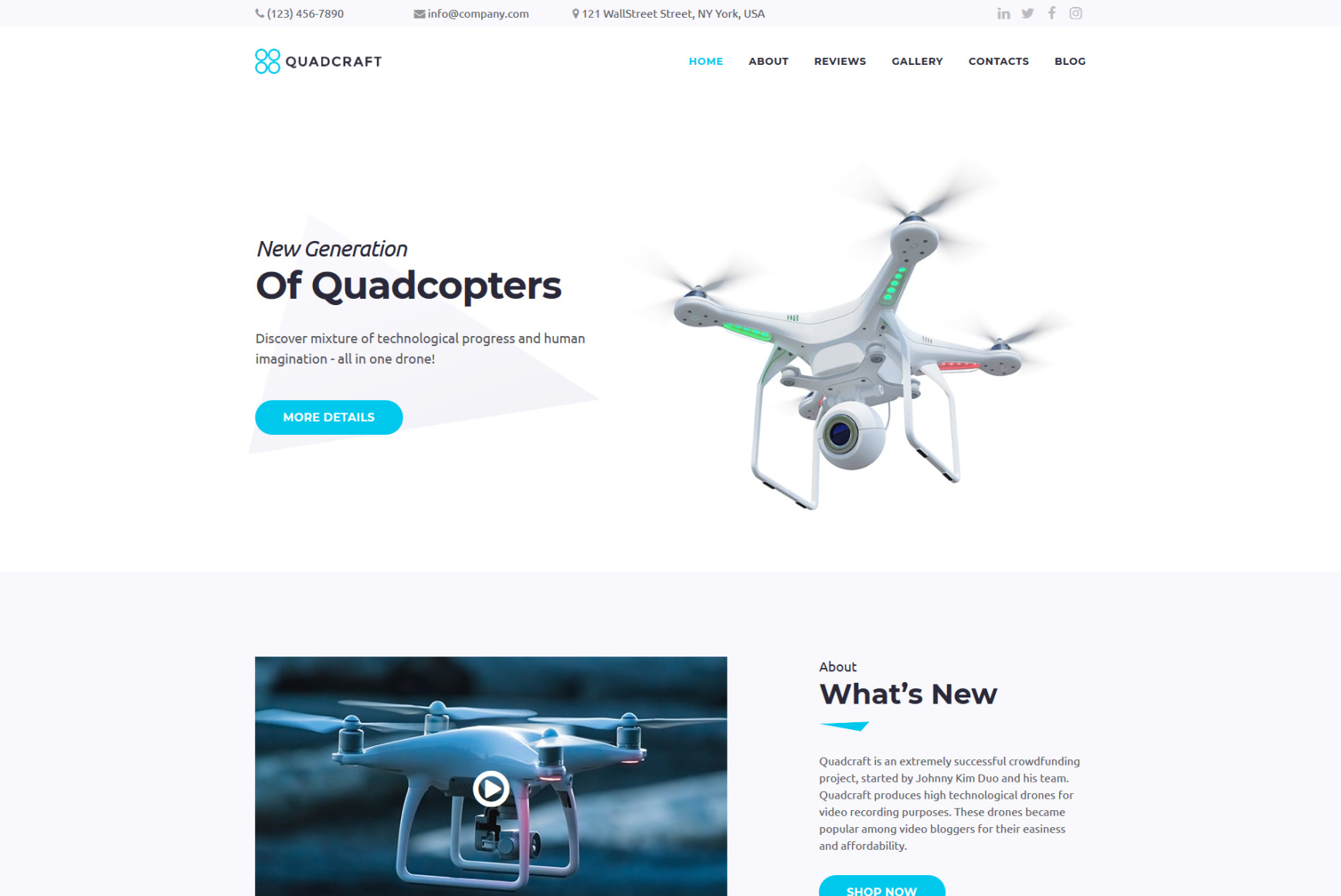This is an image of a website mock-up that appears quite generic at first glance but contains detailed information. In the upper left corner, there is a telephone icon accompanied by the number 123-456-7890, identifying it as a mock-up. An email icon resembling an envelope directs to info@company.com, and a map pin icon indicates the address 123 Wall Street, New York, New York. Social media logos for Indeed, Twitter, Facebook, and Instagram are displayed at the top.

Prominently, the brand name "QuadCraft" is displayed in capital letters to the right of four teal circles arranged in a box shape, representing the logo. The navigation menu includes tabs for Home, About, Reviews, Gallery, Contacts, and Blog, with "Home" highlighted in teal while the others remain black.

Below the menu, there is an image of a white DJI drone with four propellers and a swiveling spherical camera at the bottom. To the left of the drone, bold text reads "New Generation of QuadCopters," with "QuadCopters" in a larger font. Below this, a brief description states, "Discover a mixture of technological precision and human imagination, all in one drone." A teal capsule button labeled "more details" invites further exploration.

Underneath, there is a screenshot from a video featuring another drone, indicated by a play button overlay. To the right of this, the sections labeled "About" and "What's New" introduce further categories of content. At the bottom edge of the image, partially visible text prompts users to "Shop Now," though it is cut off.